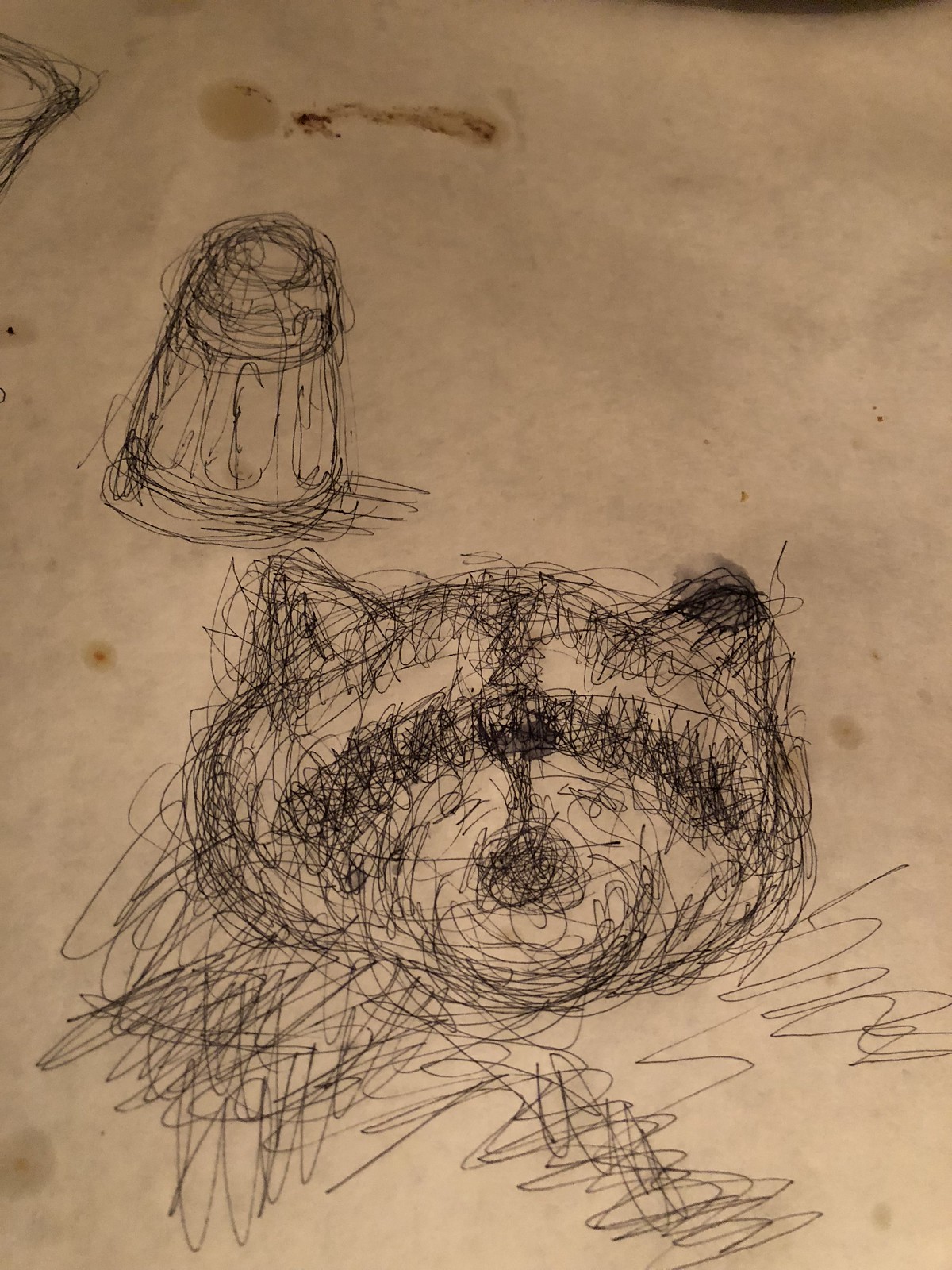In the image, a drawing on a grease-stained, off-white butcher block paper, likely from a restaurant, showcases a roughly scribbled raccoon face at the bottom. The raccoon has distinct pointed ears, a black nose, and a characteristic black stripe across its eyes, resembling a mask. Above the raccoon's face is a scribbled depiction of a shaker, possibly containing salt or pepper. The background features several additional random scribbles, further contributing to the casual, spontaneous feel of the artwork. The greasy stains scattered across the paper hint at its utilitarian use in a dining setting.